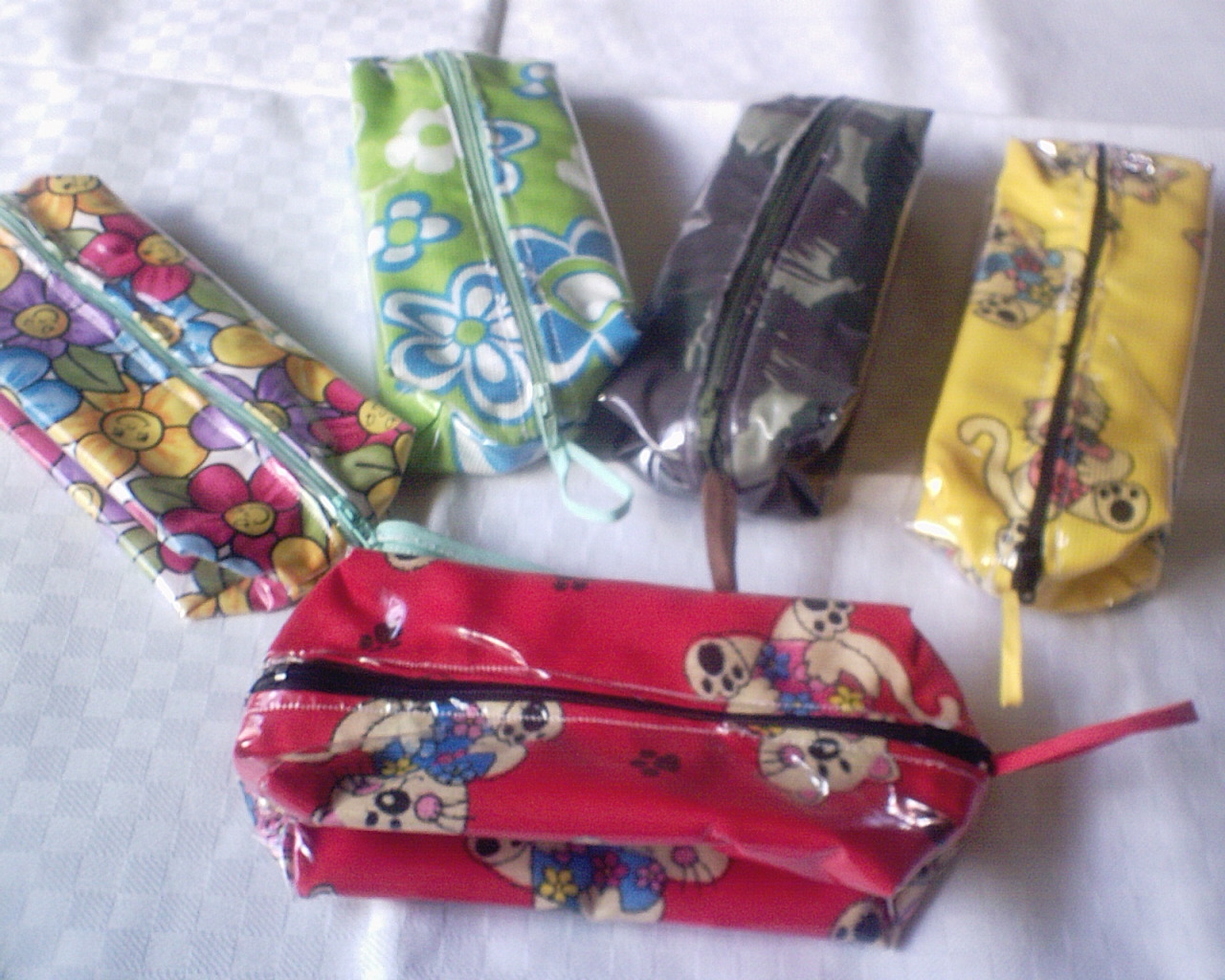This photograph shows an arrangement of five colorful zippered soft cases, likely used for makeup or as pencil cases, laid out on a white, textured cloth backdrop. The cases, made from somewhat faded fabric with vintage 70s-inspired patterns, are positioned in a fan shape with four arranged vertically and one laid horizontally at the bottom of the fan. The closest case is red, featuring a print of cats holding hearts. To the left of it is a case with whimsical, colorful flowers with faces on them. Adjacent to that is a green case adorned with blue and white flowers. Another case to the right displays a camouflage pattern. Lastly, the yellow case at the bottom of the arrangement mirrors the red one with a similar design of cats holding hearts. The background consists of a gray and white checked tablecloth, appearing as though two cloths are layered, adding texture to the setting.